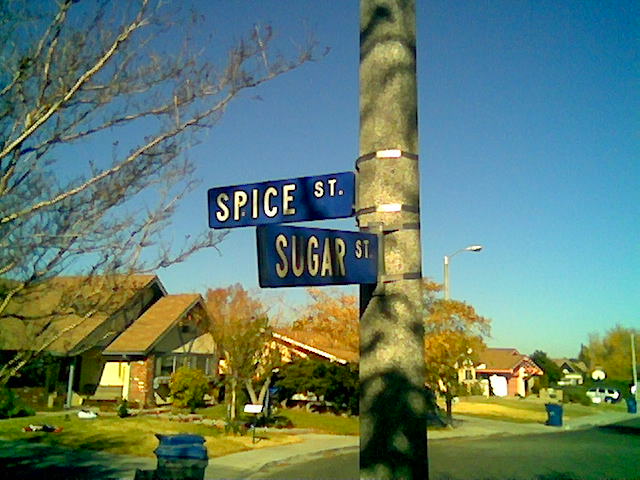This detailed photograph captures two intersecting street signs mounted on a cement pole amidst a residential neighborhood. The street signs, both blue, point in different directions: the top one, directed west, is labeled "SPICE STREET" in bold, white capital letters; the lower sign, pointing south, bears the name "SUGAR STREET" in the same style. The scene suggests a serene residential area, highlighted by a leafless tree emerging from a front yard on the left, likely indicating a fall, winter, or early spring setting. Brick houses line the street, running from the bottom left of the frame towards the middle right, providing a sense of community and structure. The curbside is adorned with streetlights, garbage cans, and recycling bins, hinting at a routine collection day. Against this peaceful backdrop, the sky stands out vividly, a flawless expanse of bright blue devoid of any clouds, enhancing the crisp and clear ambiance of the photograph.